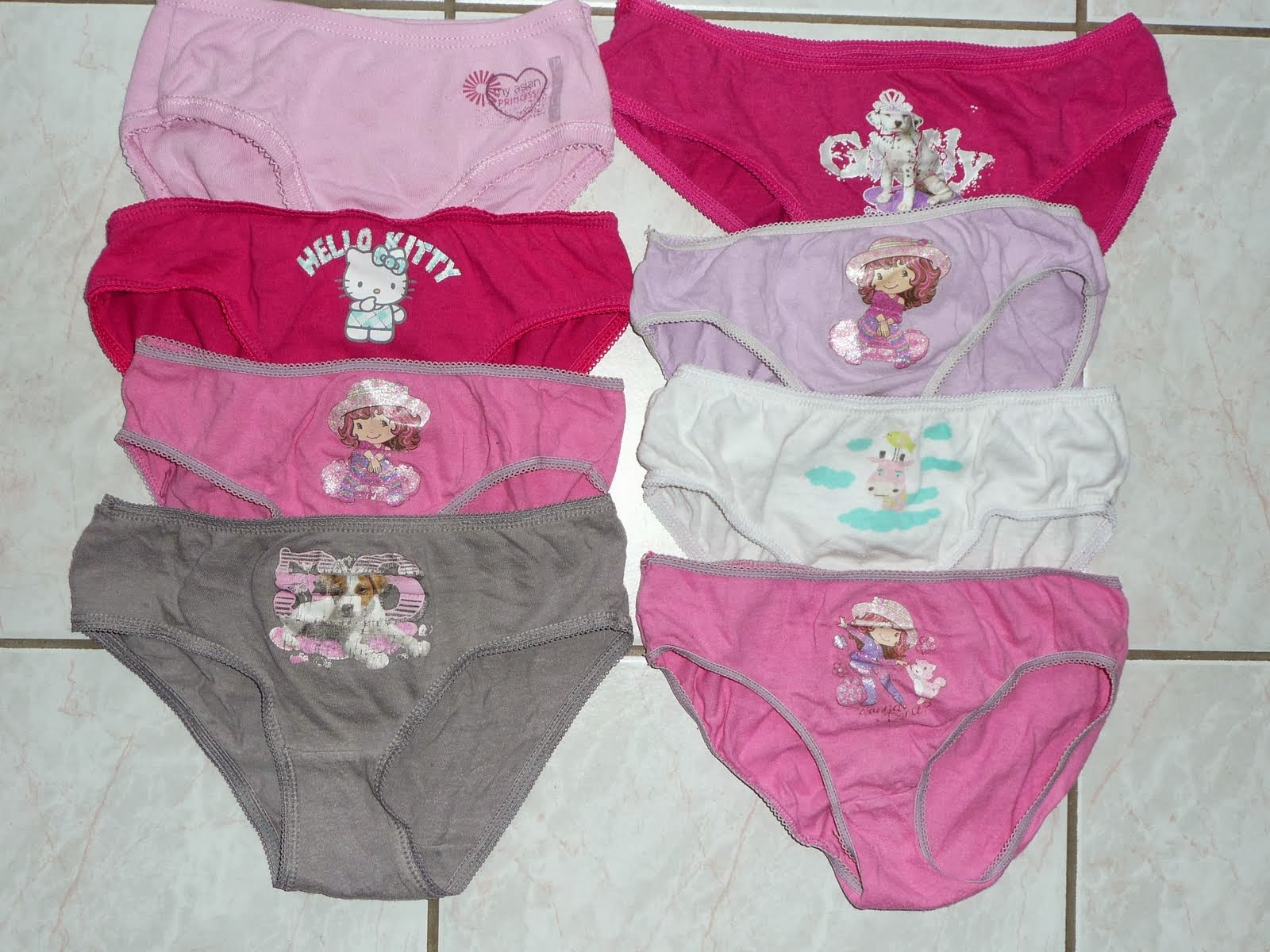The image is a digital photo taken indoors from an overhead angle. It features a white tile floor with dark grout lines, arranged in a visible grid pattern. On the floor, there are two rows of four pairs of young girls' panties, slightly overlapping but still displaying their designs clearly. The colors of the panties vary, including shades of pink, dark pink, white, gray, and lilac purple. Several pairs feature familiar characters and designs, such as Hello Kitty, Strawberry Shortcake, and a dog with white and brown spots, possibly a Dalmatian. One pair has a simple heart design in the corner. The arrangement suggests they were intentionally lined up for a photo, possibly to showcase or sell them. There are no additional writings on the screen apart from the branding on the Hello Kitty panties.